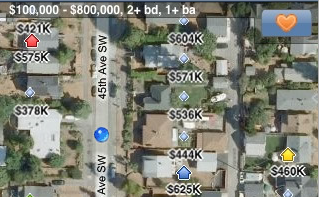An aerial view of a suburban neighborhood, likely captured from an aircraft or a drone, resembling imagery often found on Google Maps. This high-resolution photo appears to be utilized for real estate purposes, possibly for listings on Zillow.com. In the upper section of the image, a digital overlay indicates property prices ranging from $100,000 to $800,000, with attributes specifying “2+ BD” (bedrooms) and “1+ bath.” The overlay includes specific price markers for individual houses in the neighborhood. Notable listings visible include a house valued at $421K, highlighted among others priced at $575K and $378K to the left of 45th Avenue Southwest, which bisects the neighborhood. Additionally, homes on the right side of this main street are marked with prices such as $604K, $571K, $536K, $444K, $625K, and $460K. Each property is distinctly labeled, providing a comprehensive view of the area's real estate market.